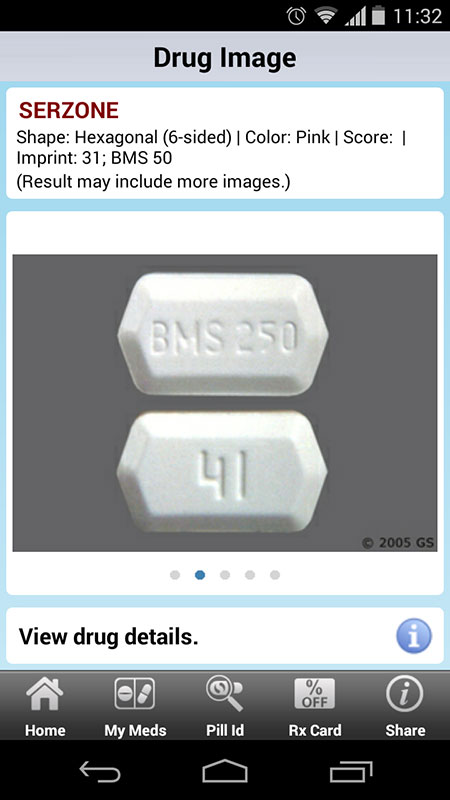This screenshot appears to be from an older Android device displaying a drug information page. The top section labeled "Drug Image" is presented in black text against a moderately desaturated blue background. Below this header, the interface shifts to a lighter, sky blue background where critical drug details are displayed.

The drug name, "Serzone," is prominently shown in red text. Directly below, detailed characteristics of the pill are provided in black text, describing a hexagonal, pink pill with a distinguishing imprint "31 BMS 50," and noting that more images may be included.

A designated white square area below this section showcases an image of the actual pharmaceutical pill. The pill is white, with one side displaying the imprint "BMS 250" and the other side stamped with "41." Both sides of the pill are clearly depicted.

Underneath the pill image, the option "View Drug Details" is presented in black text. At the bottom of the screen, a navigation bar contains five buttons labeled "Home," "My Meds," "Pill ID," "RX Card," and "Share." Additionally, three standard Android system buttons are visible near the bottom of the device interface.